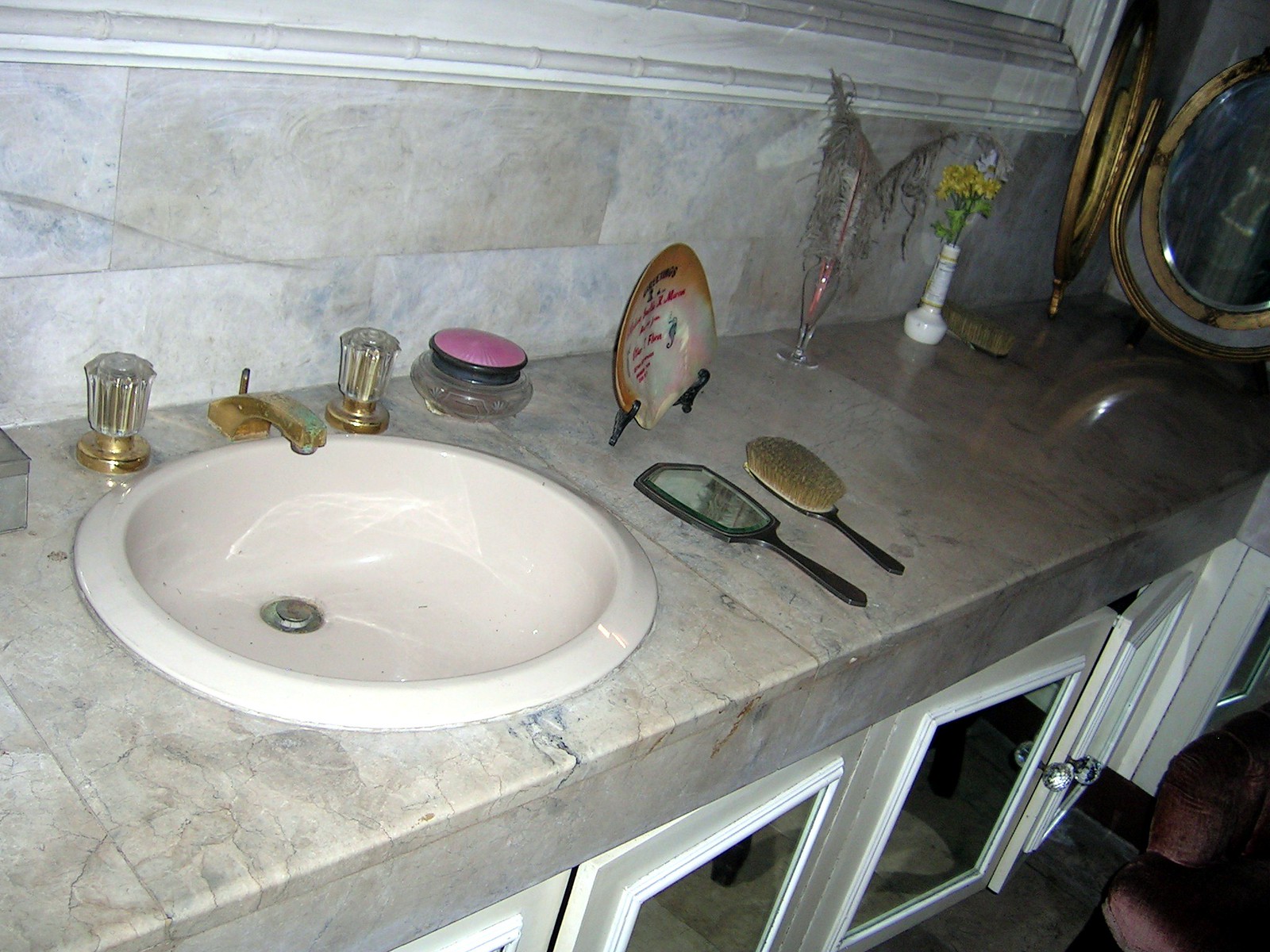This photograph captures an elegant bathroom sink area, showcasing a harmonious blend of modern fixtures and classic design elements. The backdrop features a stunning tiled wall, possibly crafted from granite, in a subtle gray hue that extends seamlessly into the countertop, creating a cohesive look. The centerpiece is a circular beige sink, complemented by a sophisticated gold faucet positioned at its center. The faucet is flanked by hot and cold handles, each adorned with a translucent, see-through plastic top set on gold bases.

To the right of the sink, a glass dish holds a curious object, black with a pink top, adding a hint of color and intrigue. Below, in the bottom right corner, lies a sleek black handheld mirror paired with a large, oval-shaped brush featuring a black handle. Above these items stands a decorative black plate stand, proudly displaying a brown oval plate with a pure white center, adding a touch of artistry and refinement.

The lower section of the image reveals mirrored cabinet doors, reflecting the serene and sophisticated ambiance of the space. This carefully curated ensemble of objects and finishes creates a bathroom that exudes both luxury and practicality.